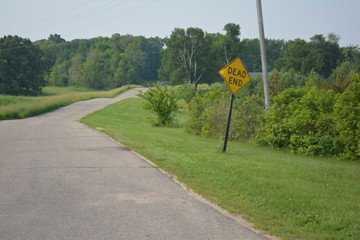The photograph captures a winding, gray stone road that meanders through a lush, green landscape. Dominating the foreground is a diamond-shaped, yellow "Dead End" sign with black text, perched on a black pole and slightly slanted to the right, positioned within a grassy and bushy area beside the road. The road itself, void of any cars, leads into a hilly terrain and seemingly ends at a dense forest, giving truth to the warning on the sign. Green bushes, plants, and tall trees densely populate the sides of the road, with an additional gray or metal pole, possibly a telephone or electric pole, jutting out from the right side. The sky above is a light blue, indicating a sunny day, enhancing the vibrant greenery and the serene, isolated nature of the road.